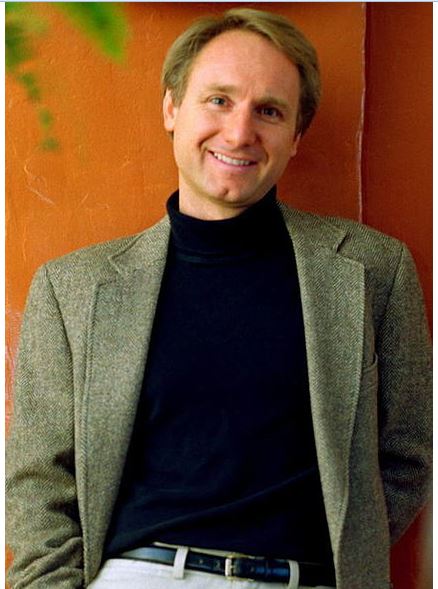This photograph showcases Dan Brown, a relatively young author, in a classic author-styled portrait seen often on book jackets. The image captures him from the top of his head to just below his belt, standing against a semi-textured, dark orange wall that might be either indoors or outdoors, with natural light streaming from the upper left corner. In the blurred upper left section of the image, some plant leaves are faintly visible. Dan Brown, a white man with short dark blonde or sandy blonde hair styled with a side part, is smiling warmly at the camera. His light eyebrows frame a clean-shaven face with attention drawn to his distinctive cleft chin. His attire consists of a tweed, wool-like blazer in a greyish-brown beige color, paired with an off-white pair of chinos or khakis, and a black leather belt featuring a gold buckle. Most notably, he is wearing a black turtleneck beneath his blazer, with one arm casually tucked behind his back, emanating an approachable yet professional demeanor typical of author photographs.